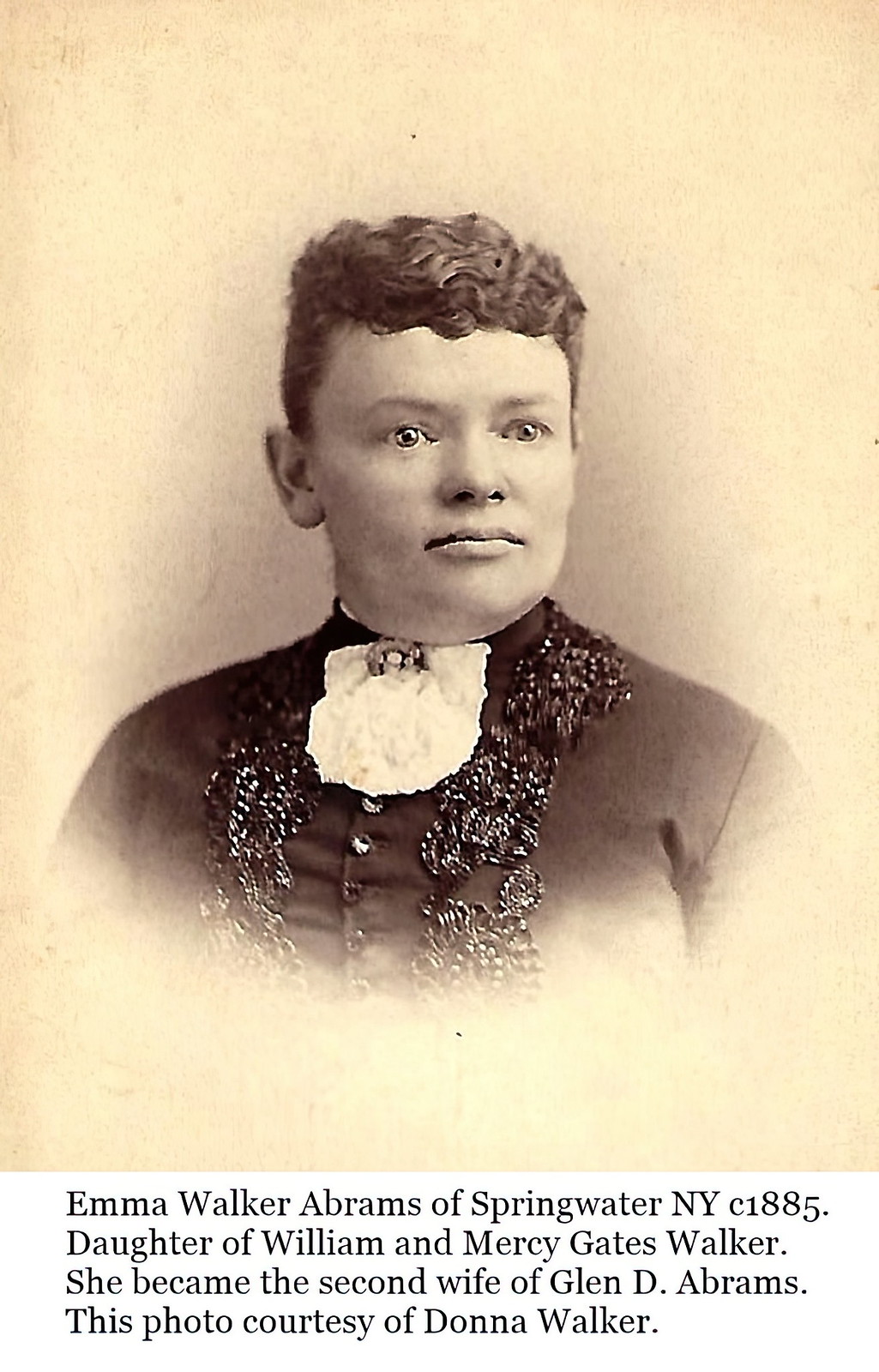This antique photograph showcases Emma Walker Abrams of Springwater, New York, circa 1885. Emma is depicted with short, curly hair, meticulously styled with the front curls pinned down and the back apparently pulled back, giving the impression of very short hair. Her gaze is directed straight at the camera, and her eyes possess a glassy, introspective quality, complemented by a neutral expression on her face. She is dressed in a dark-colored button-down dress adorned with a white, ruffled collar. The dress features an intricate floral applique design running down its front, adding a touch of elegance to her attire. The caption identifies her as the daughter of William and Mercy Gates Walker and notes how she later became the second wife of Glenn D. Abrams. This photograph is provided courtesy of Donna Walker.